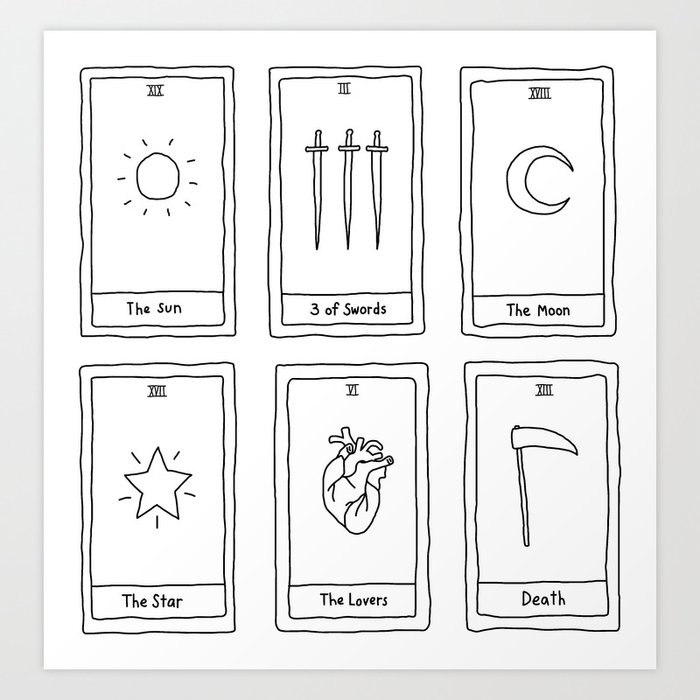This is a black-and-white illustration featuring six tarot cards arranged in two rows of three. Each card occupies a white background and displays a simplified, hand-drawn image in black ink. The cards are:

1. **The Sun**: Depicted with a straightforward illustration of the sun, complete with rays.
2. **Three of Swords**: Shows three parallel swords pointing downward.
3. **The Moon**: Features a crescent moon with the opening facing right.
4. **The Star**: Includes a five-point star emitting radiating lines to indicate it is glowing.
5. **The Lovers**: Displays an intertwined, anatomically accurate heart symbolizing the lovers.
6. **Death**: Portrays a reaper's scythe.

Each card has a Roman numeral at the top, an illustrative image in the center, and the name of the card written at the bottom, separated by a line. The entire composition is simplistic and lacks shading, with slightly wavy lines suggesting a hand-drawn, print-like quality. This artwork illustrates the essence of tarot cards without the intention of them being used as actual cards, serving instead as a representation.